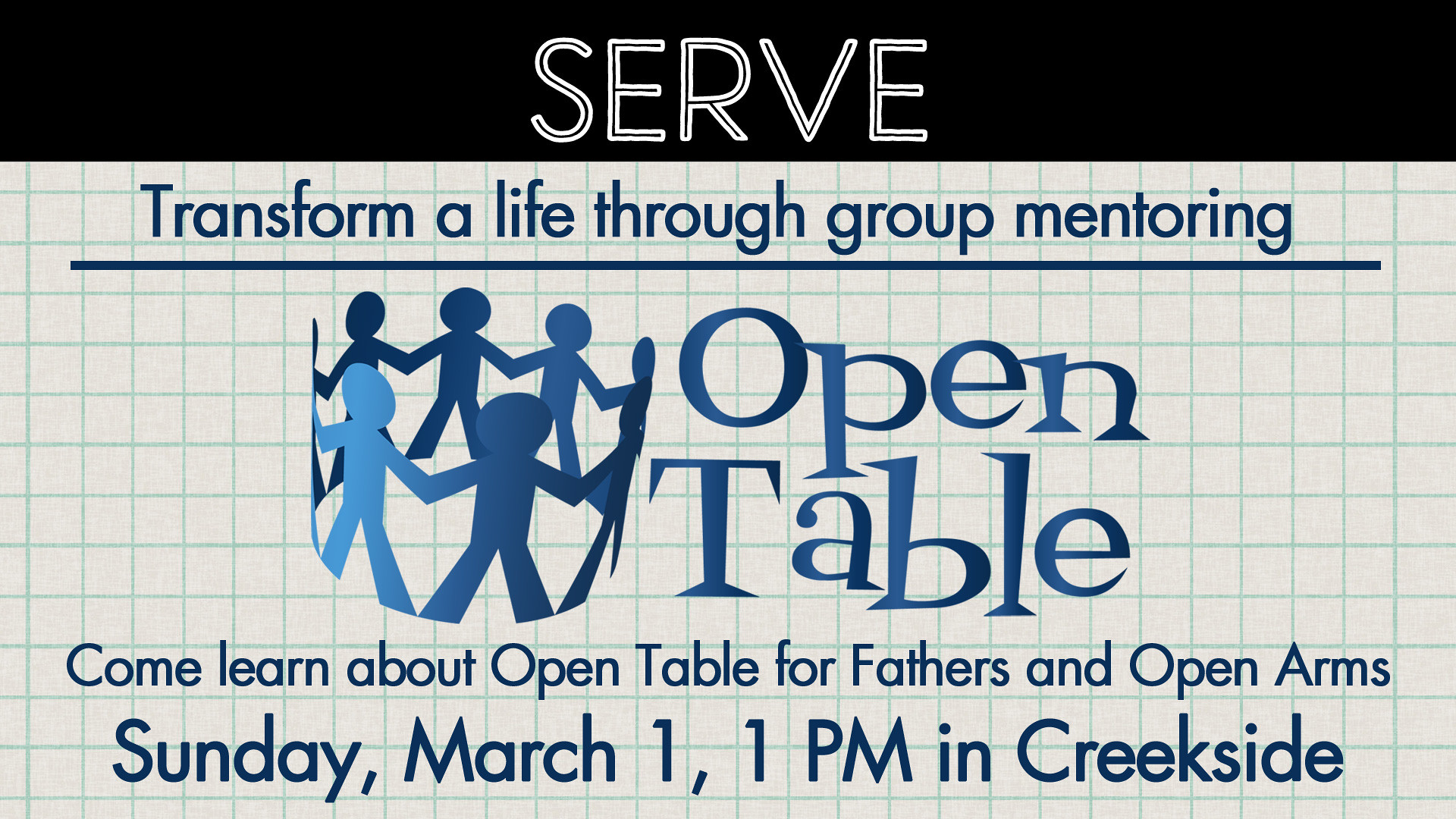The image is a detailed promotional flyer or scanned handout, likely originating from a screen grab. It features an invitation for an event called "Open Table." The background resembles graph or metric paper, providing a structured layout. At the very top, there's a black horizontal bar with the word "SERVE" in bold, white capital letters. Below this, in blue ink, the text reads, "Transform a life through group mentoring," underlined with a black line. Centralized beneath this is a logo depicting cut-out figures holding hands in a circle, reminiscent of paper snowflakes. Next to the logo, the stylized text "Open Table" is displayed. Clearly written below the logo are the words, "Come learn about Open Table for Fathers and Open Arms." At the very bottom, the flyer states in bold text, "Sunday, March 1st, 1 PM in Creekside." No additional specifics about the year or the location of Creekside are provided.